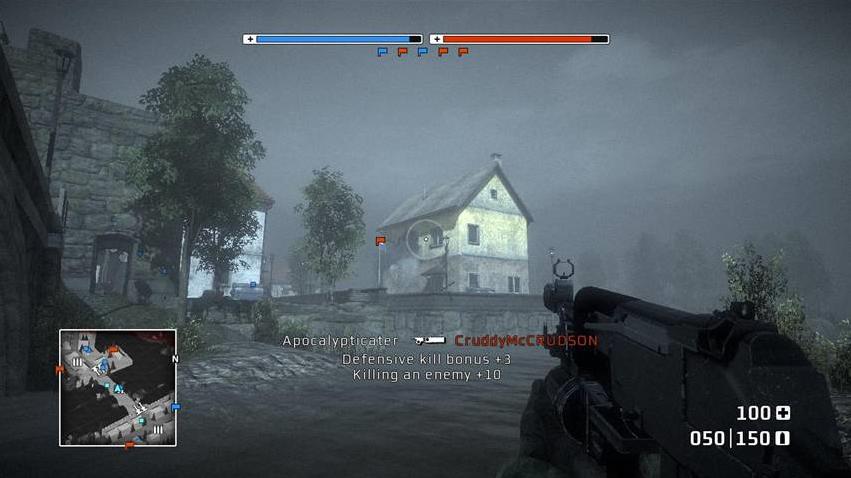This detailed image is a screenshot from a realistic-looking video game, predominantly in gray tones. On the left side of the scene, there is an old stone building with a small window and a tree with green leaves in front of it. Next to this is a white building partially obscured by another tree. Further along, there's a complete view of a second white building lined with concrete, featuring a gray peaked roof and some red detailing near the back, perhaps a marker or indicator. The sky is misty and overcast, adding to the overall gray and somber atmosphere.

In the foreground and from a first-person perspective, there's a silver and gray rifle, which resembles an MP44, extending from the bottom right corner of the screen. The rifle has a circular sight at its end. In the bottom right corner of the interface, it displays "100" next to a health symbol and "050/150" next to a bullet symbol, indicating ammunition status. 

There is white and red text across the middle of the screen that reads "Apothecator, Cruddy McFudson, defensive kill bonus +3, killing an enemy +10.” A blue bar and a red bar at the top of the screen likely denote team scores in a Capture the Flag game mode. Additional annotations include a small square map in the lower left corner, which shows the player's location with a cyan pin, team flags with red and blue pins, and other gameplay icons. The player appears to be standing in a body of gray water, further enhancing the murky and grim setting of this screenshot.